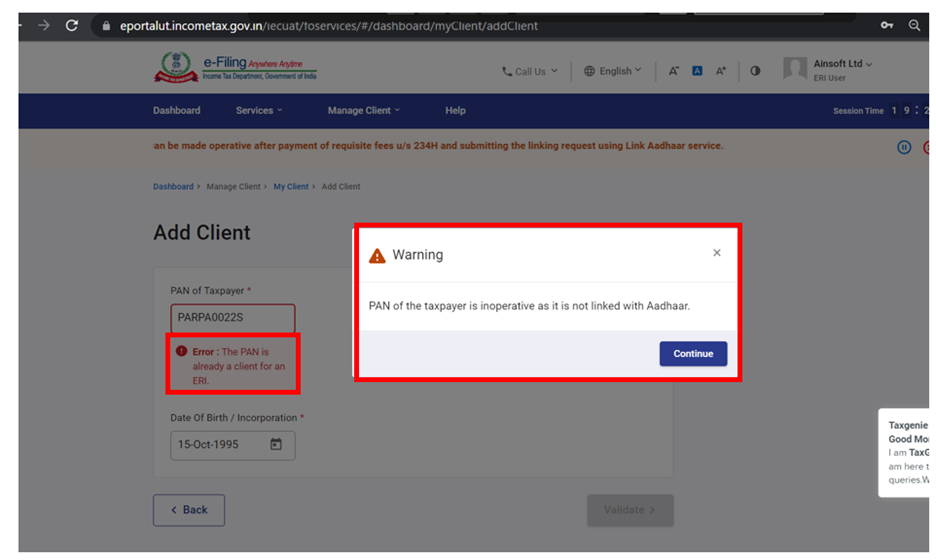This is a detailed screenshot from an e-filing website, specifically from the Tax Department's online portal at eportalut.incometax.gov.in. The image prominently features a warning pop-up with a red triangle and exclamation point, alerting the user that the PAN (Permanent Account Number) of the taxpayer is inoperative because it is not linked with Aadhaar. The red-bordered alert offers a blue 'Continue' button for the user to proceed. 

To the left of the warning, the taxpayer's PAN is shown as P-A-R-P-A-0-0-2-2-S, along with an error message stating: "The PAN is already a client for E-R-I." The taxpayer's date of birth or incorporation is listed as 15 October 1995. The entire alert is a crucial reminder for users to link their PAN with Aadhaar to ensure the operability of their tax documentation.